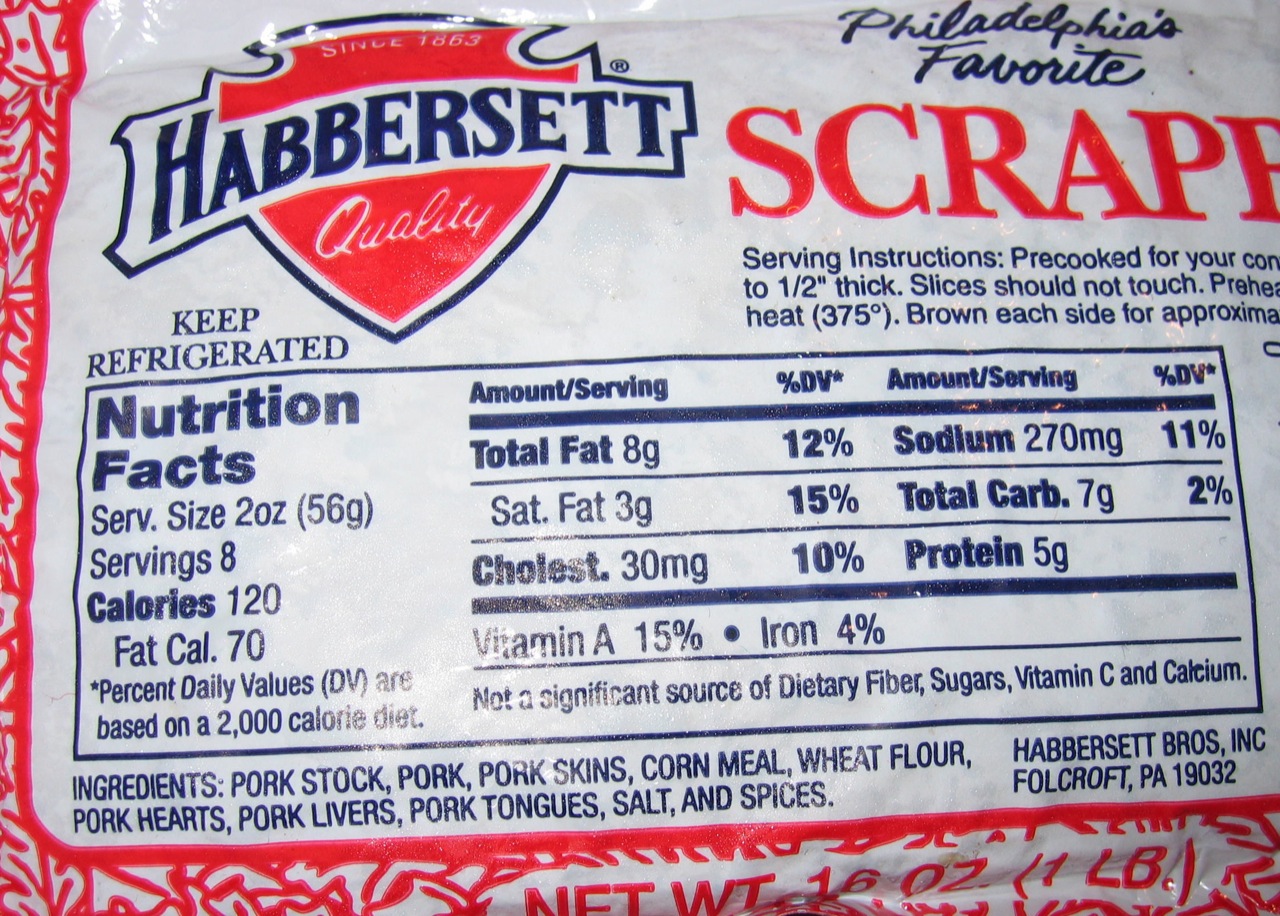The image is a landscape-format, color photograph showcasing the back of a packaged food product from Habbersett Quality, a brand established in 1863. Prominently featuring Philadelphia's Favorite Scrapple, the white-background packaging has a reddish-colored border at the left and bottom edges. In the top-right and left-top-middle sections, the text "Philadelphia's Favorite Scrapple" and "Since 1863 HABBERSETT Quality" respectively, are displayed, with the latter framed within a badge-like red structure. The product is labeled "NET WT 16 oz (1 lb)" at the bottom right.

The central portion of the image highlights a large rectangle containing detailed Nutrition Facts, which indicate that a serving size is 2 oz (56g) with 8 servings per container. Key nutritional values include 120 calories per serving with 70 calories from fat, 8g total fat, 30mg cholesterol, 70mg sodium, 7g total carbohydrates, and 5g protein. Vitamins and minerals like Vitamin A and iron are also listed.

Additionally, ingredients are detailed, consisting of pork stock, pork, pork skins, cornmeal, wheat flour, pork hearts, pork livers, pork tongues, salt, and spices. Serving instructions suggest the product is pre-cooked and recommend slicing it up to one inch thick. The package emphasizes the need to keep the product refrigerated. The text throughout the image is presented in a combination of dark blue and red colors, giving a clear and distinctive visual contrast. The photo appears to be taken indoors.